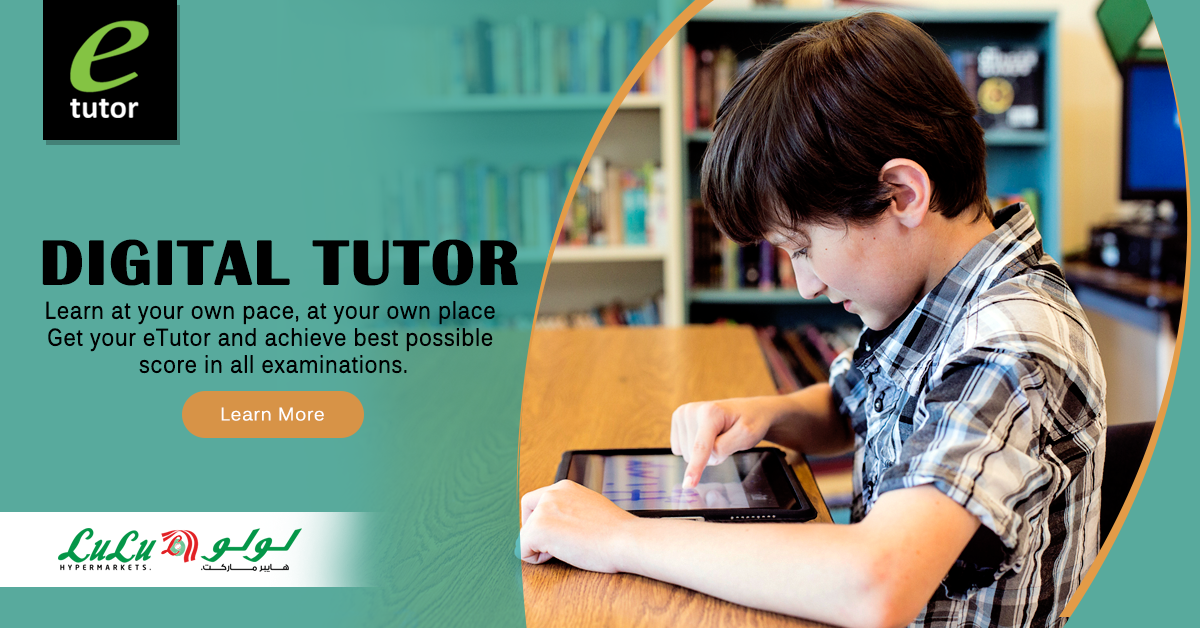The advertisement for the Digital Tutor software is presented in a long, horizontal rectangular image divided into two sections. The left side features a solid aqua green background with the e-tutor logo in the upper left corner. The logo showcases a lowercase "e" in green and the word "tutor" in white below it. Below the logo, prominent black text reads "Digital Tutor" followed by the tagline: "Learn at your own pace, at your own place. Get your e-tutor and achieve the best possible score in all examinations." Below the tagline, there is an orange button labeled "Learn More."

On the right side of the image, a photograph depicts a young boy with short brown hair, wearing a black, white, and gray plaid short-sleeve shirt. He is seated at a table in what appears to be a library or classroom, surrounded by numerous books. The boy is engaged with a tablet, likely using the Digital Tutor software. The overall background on the right side peacefully blends into the left, creating a cohesive and engaging visual for the advertisement aimed at promoting e-tutoring services for academic excellence.